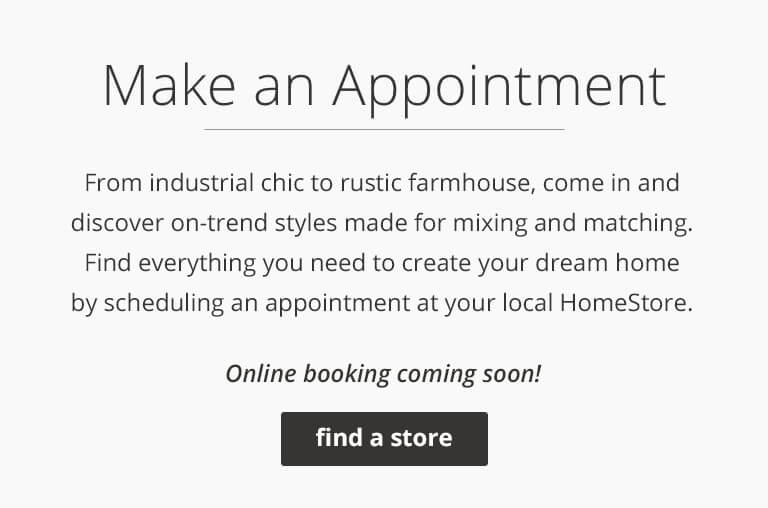On a grayish background, the focal point of the image is a bold, black text at the top reading "Make an Appointment". Directly beneath this is a centered, but narrowly extended, thin black bar. The following text below this bar reads: "From industrial sleek to rustic farmhouse, come in and discover endless styles for mixing and matching. Find everything you need to create your dream home by scheduling an appointment at your local home store." Further down in the center of the image, in bold black text, it announces, "Online booking coming soon!" Towards the bottom, a black rectangle contains the phrase "find a store" in all lowercase white text. This streamlined design focuses on promotional details and service announcements for a home store.